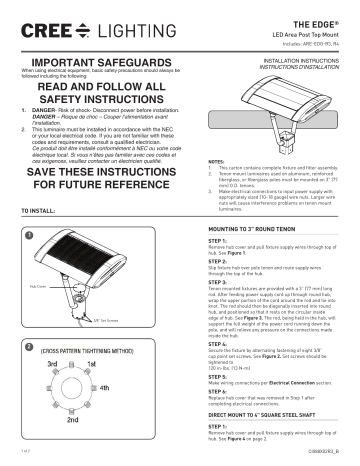The image depicts a detailed installation guide for an outdoor LED lighting system. The centerpiece of the guide highlights a vibrant, softly lit LED setup intended for edge lighting. Several components of the lighting system are shown, including safeguards for weatherproofing, such as protection against rainfall. Safety instructions are prominently outlined, warning about potential dangers and providing detailed steps for secure installation.

The installation process is broken down into a methodical sequence, emphasizing a cross pattern tightening technique. The instructions detail:
1. Starting with the first mount point at the top right.
2. Moving to the second at the bottom.
3. Continuing to the third at the top left.
4. Finishing with the fourth on the right.

Each step is clearly labeled from Step One to Step Five, making it easy to follow along. The guide also includes various text labels to highlight key areas and components. This comprehensive descriptive outline ensures that even those unfamiliar with the setup can successfully install and utilize the LED lighting system safely and effectively.